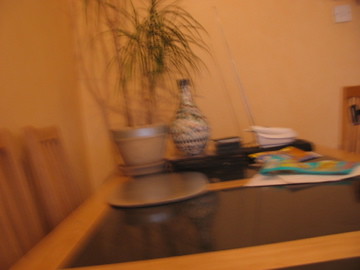The blurry image depicts a dining room featuring a wooden dining set against peach-colored walls. The rectangular table has a brown wood outline and a black center. There are at least two wooden chairs with straight backs and slats on the left and possibly one more on the far right. On the tabletop, there is a beige planter with silver trimming, containing long brown stems and green fern-like leaves. Additionally, there's a yellow vase adorned with blue flowers, a black object, some turquoise and white papers, and a white ceramic bowl, possibly oval in shape, located in the background. The dining table also holds a beige and brown vase with horizontal squiggly patterns. A light switch can be seen in the upper right corner of the peach-colored wall.